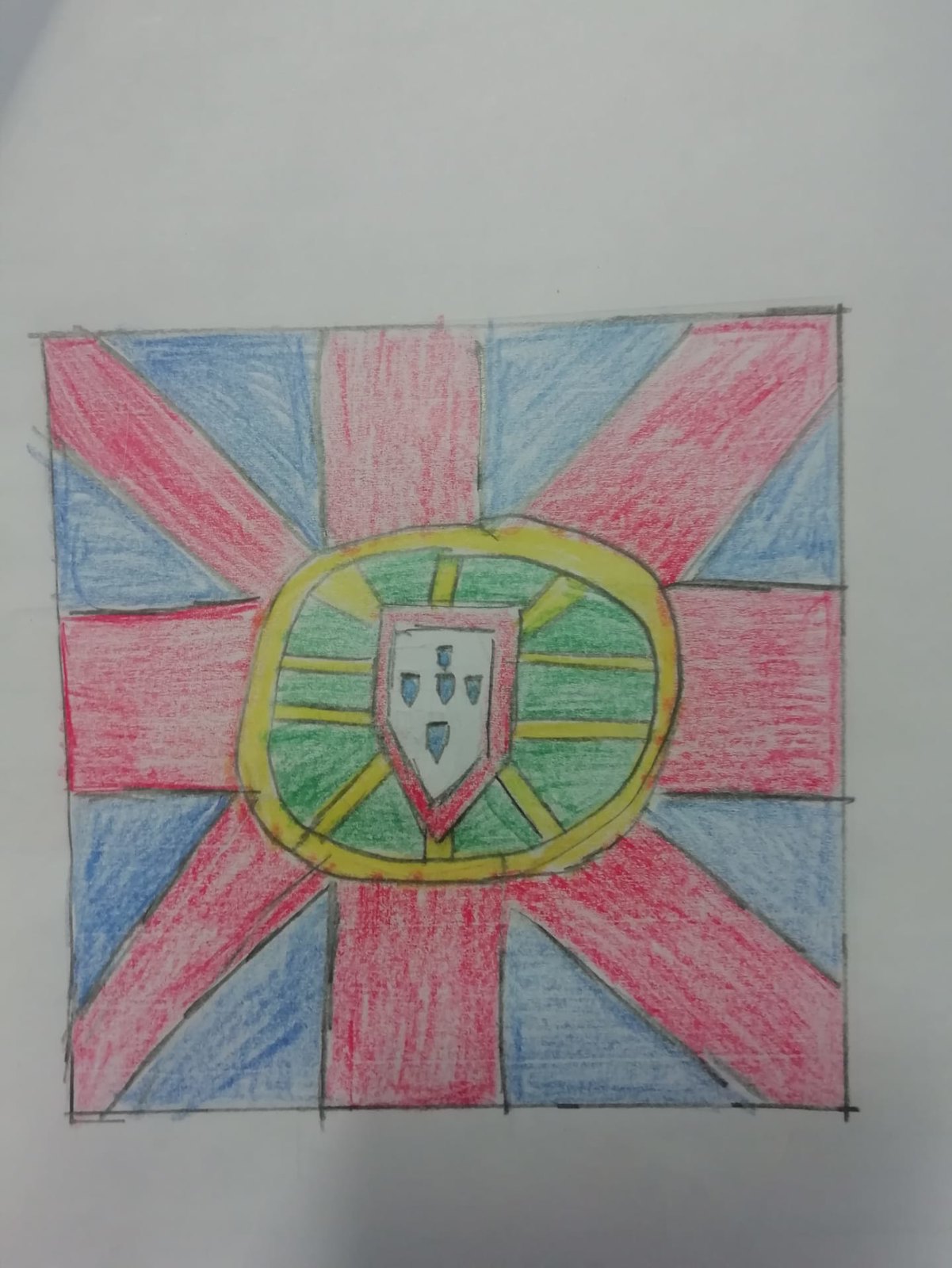This image features a slightly cropped, off-white or gray-toned sheet of paper, particularly in the upper left corner where it appears to be folded back, contributing to its gray appearance. The focal point of the image is a colorful geometric design taking up most of the page. The design is dominated by a box with a deep blue background interspersed with red stripes. A prominent red cross lays over the blue backdrop, which is further intersected by another red 'X', reminiscent of certain national flags.

Within the center of this cross arrangement is an oblong shape, which seems to be intended as a circle but appears more oval due to its freehand design. This shape is outlined in black and encircled by a thick yellow line. Additional details include two horizontal yellow lines running across the center of the image, along with a vertical yellow line also positioned centrally.

At the very core of this elaborate design is an overlay featuring a shield with a red border and a white face. Inside this central shield, there are three smaller shield icons aligned in a row and two additional small blue shield icons, one positioned above and one below the central shield, adding layers of intricate detail to the composition.